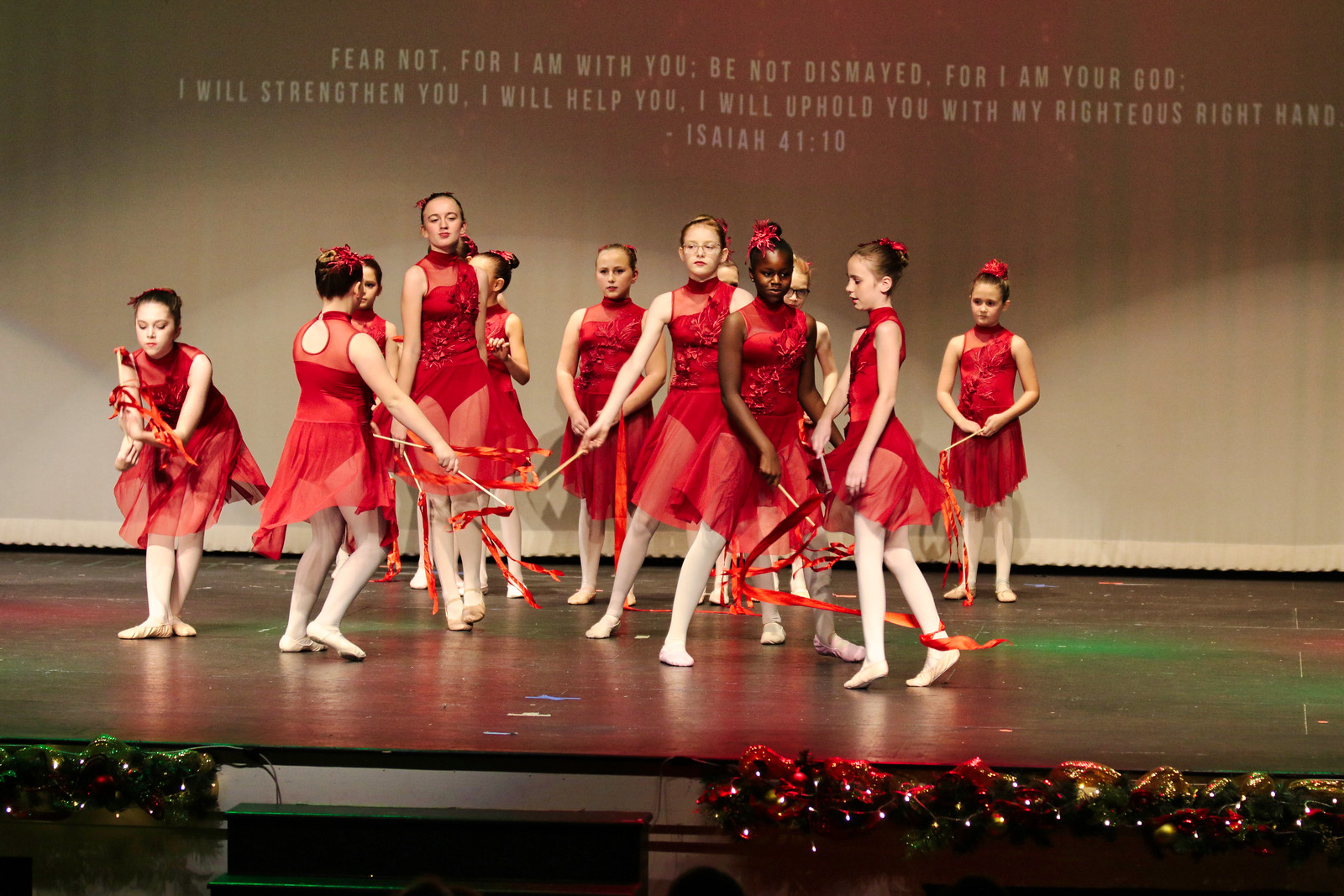In this photograph, a group of around 12 young girls is captured performing on a stage, possibly during a Christmas production. They are adorned in red ballet dresses with sheer skirts, white tights, and beige ballet shoes. Each girl holds a white stick adorned with red ribbons. The stage is decorated with lighting and garlands along the front. The backdrop features a white wall with a dark brown floor. Above the performers, text is displayed, reading, "Fear not, for I am with you. Be not dismayed, for I am your God. I will strengthen you, I will help you, I will uphold you with my righteous right hand." Isaiah 41:10. The scene is vibrant and dynamic, with the girls in motion, not in a straight line but rather spread out in an animated formation.